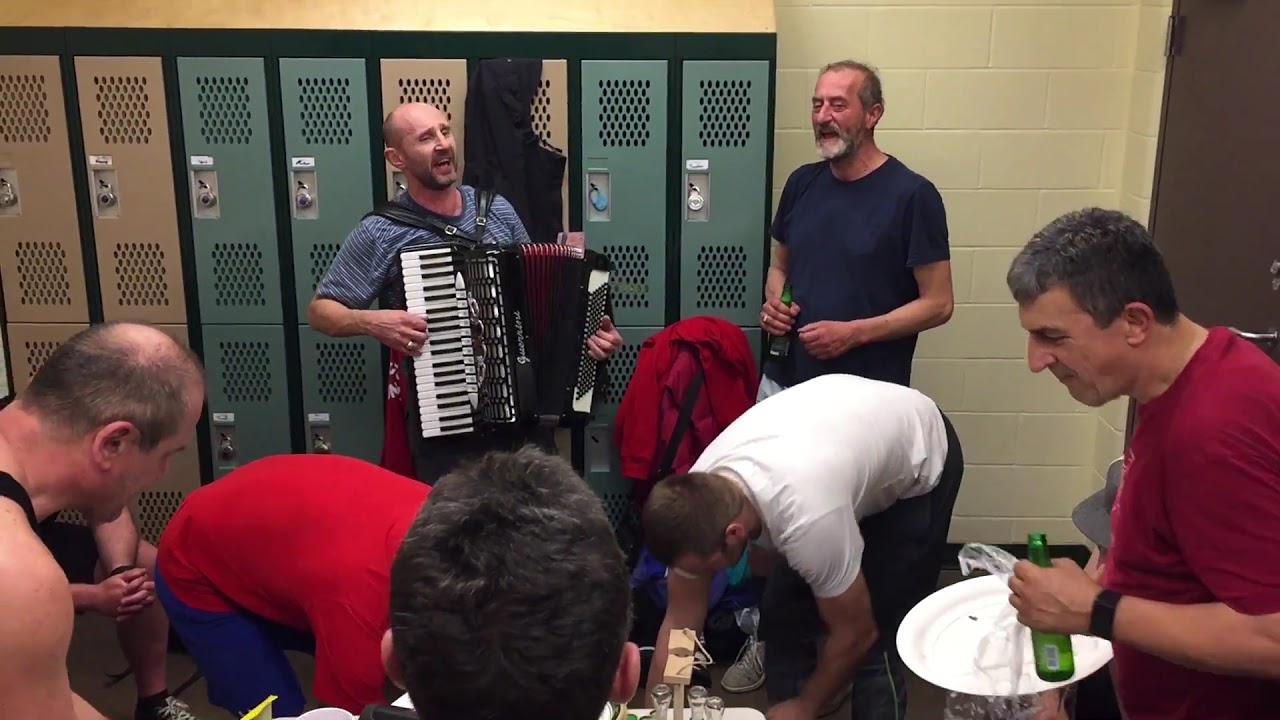The image showcases a lively scene in a men's locker room with a yellow-painted cinderblock wall backdrop. The room features two levels of lockers, with the upper row predominantly greenish-blue and the lower row tan or silver. Around seven or eight men are present, engaged in various activities. Central to the image is a man in a short-sleeved, blue-striped shirt playing an accordion, his mouth open as if singing. To his right stands an older gentleman with a gray beard, wearing a navy blue shirt and holding a green bottle of beer, seemingly singing along. At the right bottom corner, another man with a maroon-red shirt holds a green bottle of beer and a paper plate, suggesting he has finished eating. Flanking these key figures are two men bent over, one in a red shirt and the other in a white shirt, possibly tending to something on the ground or a table, which is out of view. The scene is filled with camaraderie and a casual, convivial atmosphere.